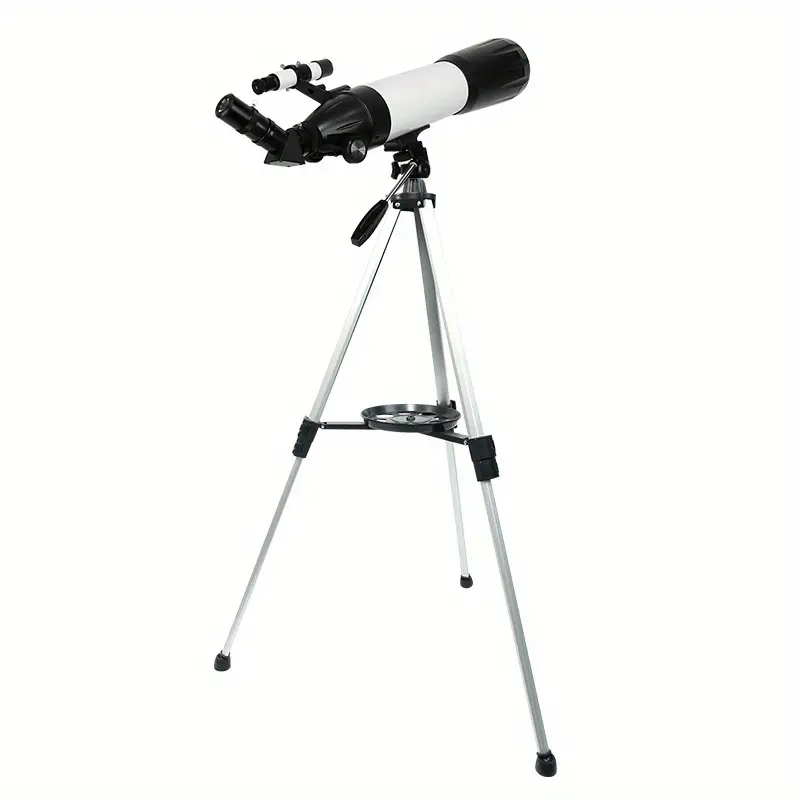The image depicts a telescope mounted on a light silver or white tripod with long, thin legs and black stands on the feet for stability. The telescope itself features a cylindrical body: the ends are black, while the central tubular section is white. A distinctive black eyepiece is angled towards the viewer. An additional smaller cylindrical scope, composed of alternating black and white sections, is attached above the main telescope. The tripod is reinforced with a central black bracing, upon which a circular silver plate is situated. Below the telescope, there is a grip or handle allowing adjustment of the view.